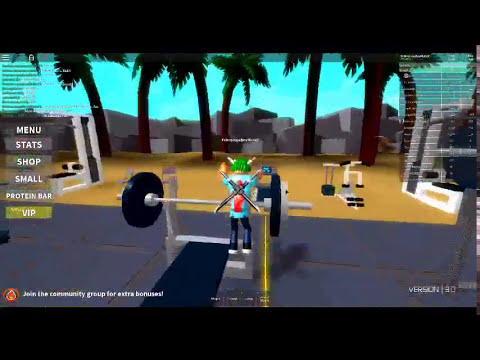This image from a video game displays a character with striking green hair and possibly white horns, wearing blue jeans and a blue shirt with red accents, and wielding two black swords on their back. Central to the scene is a weightlifting setup with a black-barred barbell loaded with black weights, situated on a black bench with a white frame. The character is positioned in front of this setup, seemingly about to engage with the weights.

Flanking the scene are various other pieces of white and black exercise equipment, including what appears to be a treadmill leading up to the weight. The background hints at an outdoor environment with a blue sky, gray mountains, tan sand, and stylized palm trees that have large green leaves and partly obscured brown trunks. Additionally, gray cube-like structures suggest the presence of distant buildings.

Text elements are prominent in the image. Along the left-hand corner, a menu appears with uppercase white letters reading "MENU, STATS, SHOP, SMALL, PROTEIN BAR, VIP," displayed on gray backgrounds, except "VIP" which is on a gold background. The bottom left corner features the message "Join the Community Group for Extra Bonuses" in white text next to a flame-like logo in red and orange within a red circle. The bottom right corner has “Version 3.0” in white letters on a gray background. This detailed setting and interface confirm that the image is from a video game, possibly a gaming app.